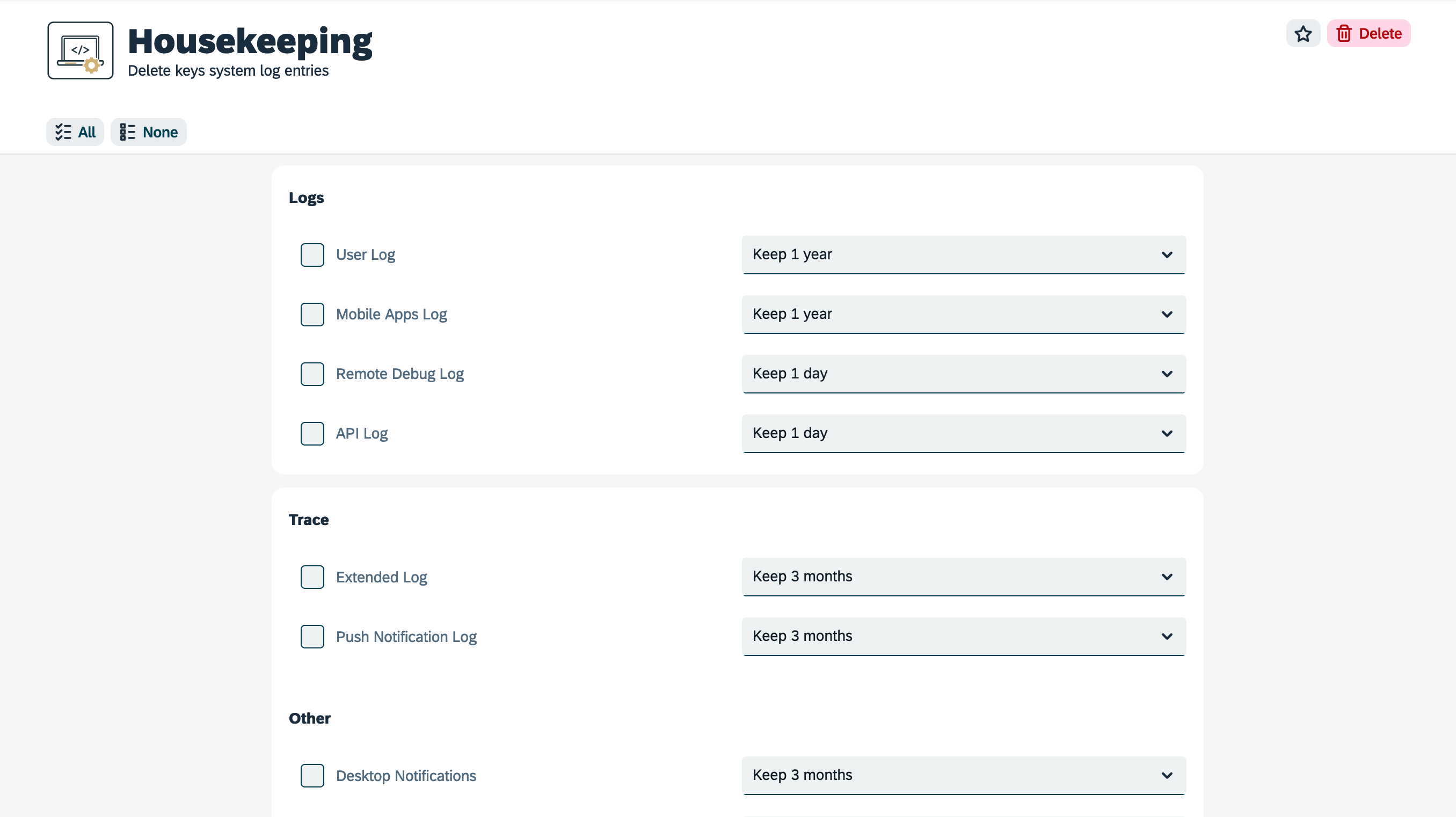In this image, we are presented with a program interface focused on log management and housekeeping tasks. In the top-left corner, a section titled "Housekeeping" addresses the deletion of key system log entries. Below this heading are several filtering options: "All" and "None."

The interface categorizes logs into various types with specific retention periods outlined for each:
- **User Log**: Retention period is set to one year.
- **Mobile Apps Log**: Retention period is also set to one year.
- **Remote Debug Log**: Retention period is restricted to one day.
- **API Log**: Retention period is similarly limited to one day.
- **Trace, Extended Log**: Retention period extends up to three months.
- **Push Notification Log**: Retention period is also designated for three months.
- **Others, Desktop Notifications**: Retention period matches that of push notifications, at three months.

The bottom portion of the page is a clean, white area providing visual separation from the detailed log settings above. In the top-right corner of the interface, there are two action buttons available: a "Delete" button for clearing selected log entries and a "Favorite" button for easy access or prioritizing tasks. The layout is designed for ease of navigation and user interaction, ensuring efficient log management.